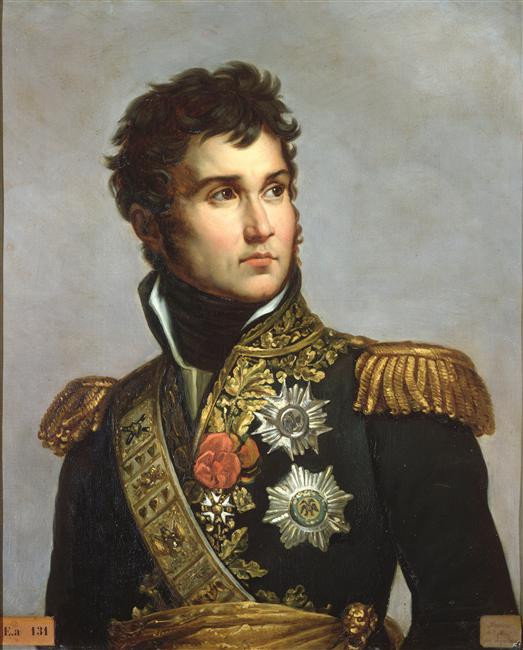This is an old-fashioned portrait painting depicting a high-ranking military general or soldier from a bygone era. The man, with curly dark brown hair and brown eyes, is attired in an elaborate uniform featuring a black coat adorned with thick, gold trim along the lapels, shoulders, and waist. His jacket is further embellished with silver star-shaped badges on the chest, suggesting his distinguished rank. The uniform also includes decorated shoulder pads with fringes and a prominent gold sash. He gazes thoughtfully to the right, set against a muted gray background, conveying a sense of leadership and authority.